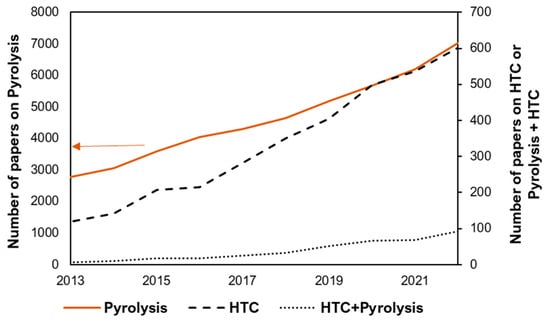The graph, depicted in black and white with an exception of an orange solid line, showcases the number of papers on pyrolysis and HTC (Hydrothermal Carbonization). The orange line, representing pyrolysis, shows a significant upward trajectory, starting just below 3000 and rising well above 600 on the right-hand side. This line stands out as the only colored element in the graph. A dotted line, indicative of HTC, begins at zero and climbs up to 100, while a heavier dashed line represents a combination of HTC and pyrolysis, starting around 1500 and also ascending, albeit less dramatically than the orange line. The left y-axis ranges from 0 to 8000 papers on pyrolysis, and the right y-axis ranges from 0 to 700 papers on HTC or the combination of both processes. The graph reflects a growing interest in research papers covering these topics, although its context and background details are not clearly explained in the image itself.